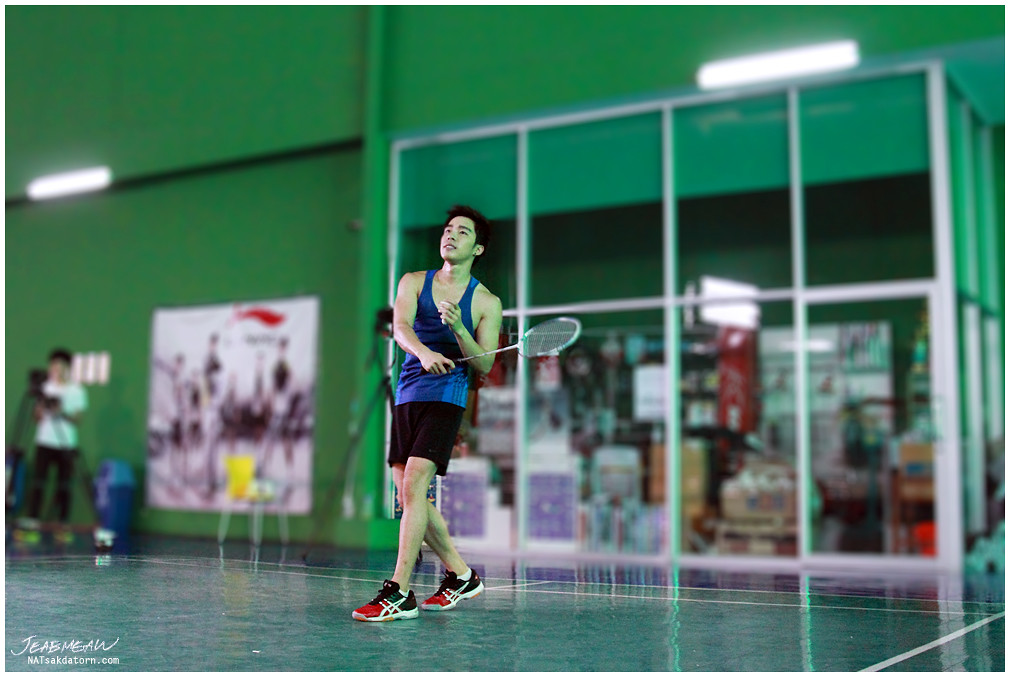The photograph captures a young Asian man playing badminton inside a gymnasium or a sports club. The athlete, situated in the center of the image, is wearing black shorts, a blue tank top, and red and black Asics sneakers. He has short black hair and is holding a badminton racquet in his right hand, which is extended across his body as if he has just swung at a birdie. His gaze is directed upwards and to the left, likely following the trajectory of the shuttlecock he just hit. 

The gymnasium features green walls and a shiny playing surface with white lines marking the badminton court. In the blurred background, there's a large white poster on the green wall and a yellow chair. Additionally, a man in black pants and a white t-shirt is standing to the left, possibly filming the match with a camera mounted on a tripod. Behind the player, the area contains glass window panes that appear to reveal a shop of some kind. A blue wastebasket is also visible near the photographer's watermark, "Jibmyaw Natsakadetorm.com," in the bottom left corner of the image.